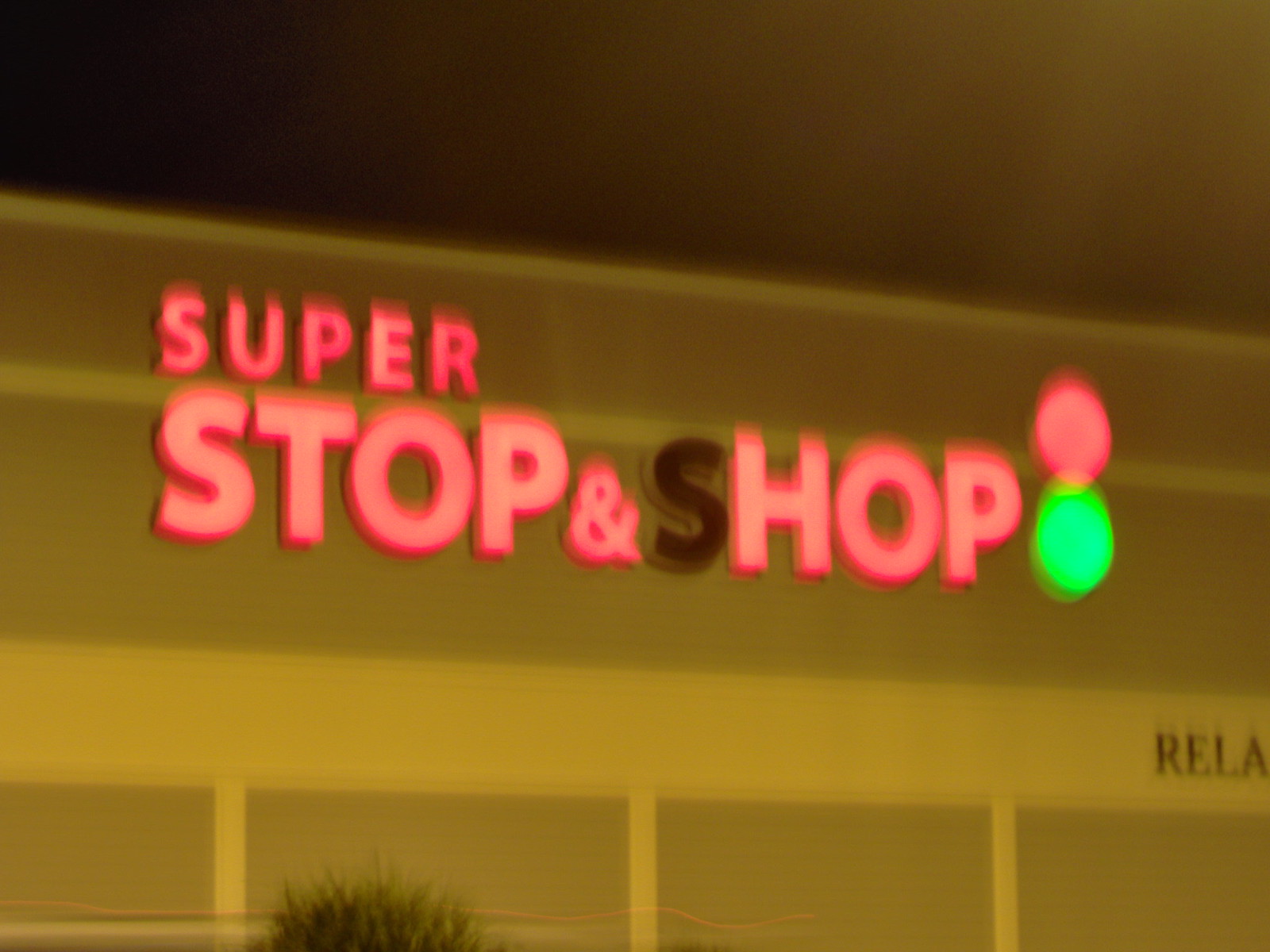The image depicts a blurry, nighttime view of a store sign mounted at the top of a building. The sign, illuminated in red, reads "Super Stop & Shop," with the word "Super" written in smaller font above the larger "Stop & Shop." Notably, the 'S' in "Shop" is not lit, appearing as a dull burgundy color, suggesting a bulb outage. Below the sign, the letters "R-E-L-A" are visible on a white strip painted on the building's wall. Adjacent to the sign are two lighted circles: the bottom one green and the top one red. The faint glow of a street light is suggested by the overall illumination and the dark, starless sky hints at the nighttime setting. At the lower left corner of the image, part of a green bush can be seen, adding a touch of nature to the urban scene.